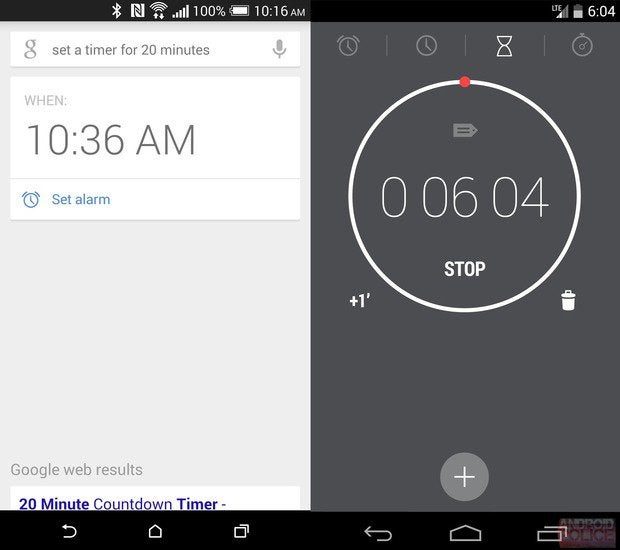Detailed Caption:

An image showcases two side-by-side smartphone screenshots displaying different sections and functionalities. 

On the top half of the first screenshot, a black status bar spans across the screen. Towards the center-left of this bar, various icons are visible in the following sequence: Bluetooth, an N-logo, Wi-Fi signal strength indicator, full cellular signal bars, a 100% battery icon, and the time reading as 10:16 AM. Far right on this bar shows partial cell coverage with LTE service, a battery icon about a quarter depleted, and the time indicated as 6:04.

The main screen area underneath the status bar has a predominantly white or light gray background, featuring a search bar with the Google 'G' logo and microphone icon. The search query reads "Set a timer for 20 minutes." Below this search bar, there is a small black strip displaying "when" followed by the time 10:36 AM in black text. This is followed by search suggestions such as "Set an alarm." Further down, a section labeled "Google Web Results" provides a 20-minute countdown timer link.

On the second screenshot, the background maintains a grayish tint featuring a set of timer-related icons: a gray alarm clock, a generic analog clock, a white hourglass, and a stopwatch. A circular interface with a red top section and centered name tag reads 06:04 (or 6 minutes and 4 seconds). Below, there are functional options including a "Stop" button, a "+1 min" button, and a trash can icon to presumably delete the timer.

At the very bottom, the screen displays navigation buttons in black, showing icons for: Back, Home, and a double-square multitasking view, appearing on both sides of the navigation bar.

This detailed screenshot is a comprehensive snapshot of the timer and search functionalities on a smartphone, providing clear insights into the user interface elements and their arrangements.